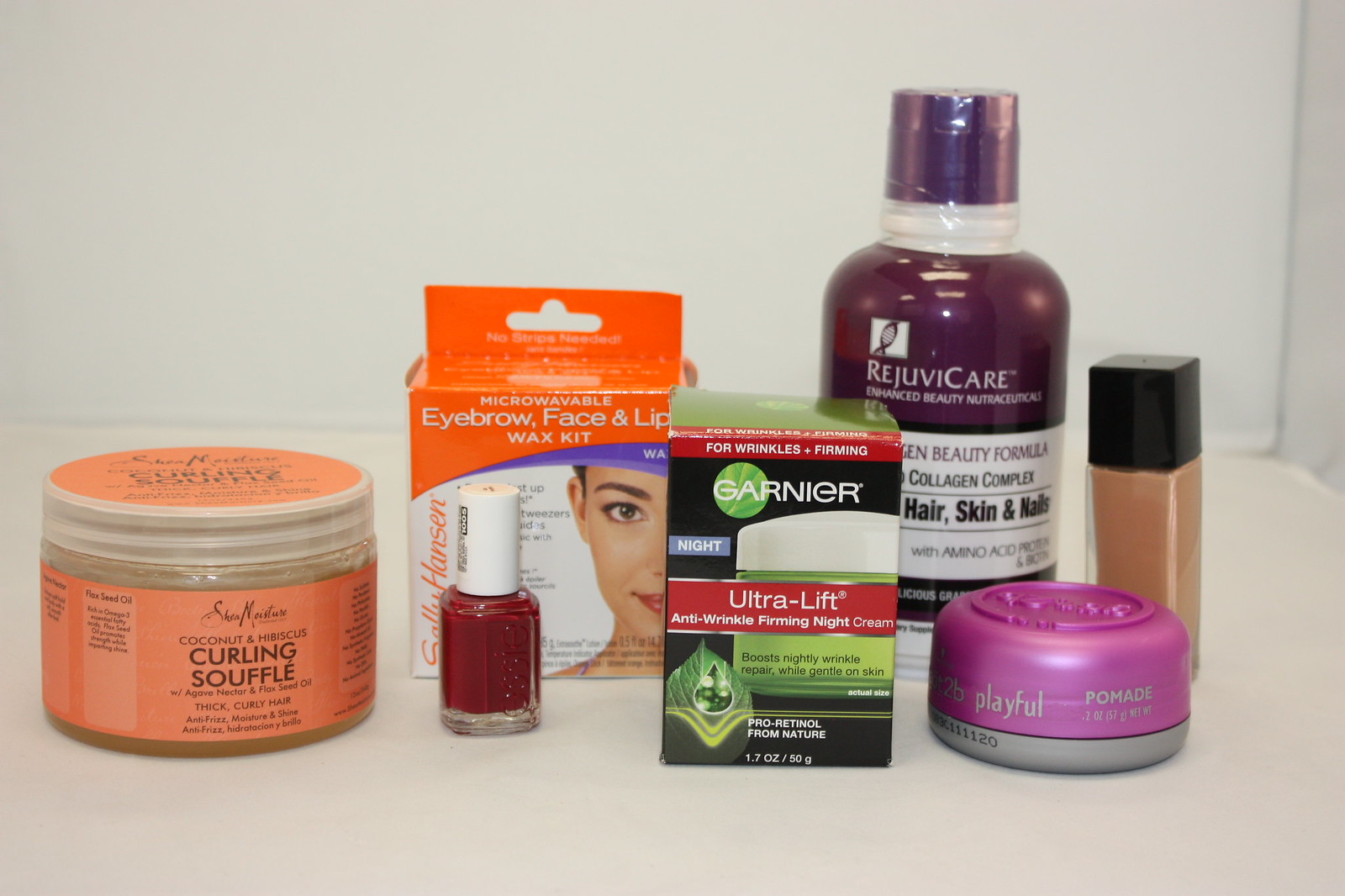This close-up image showcases a meticulously arranged collection of seven beauty products on a pristine white table surface.

Starting from the left, there is an orange jar of Shea Moisture's Coconut & Hibiscus Curling Soufflé, known for enhancing natural curls. Next to it, in a small orange and white box adorned with a facial graphic, is a microwavable eyebrow, face, and lip wax kit.

In front of this wax kit box, a vibrant red bottle of nail polish stands elegantly, catching the light. Adjacent to the wax kit, there is a striking black, red, and green package of Garnier Ultra Lift Anti-Wrinkle Firming Night Cream, promising to rejuvenate skin overnight.

Moving further right, a sleek purple and white bottle labeled Rejuve Care Advanced Beauty Nutraceuticals offers supplements designed for healthier hair, skin, and nails. Following this, a cute, rounded purple cylinder jar marked "Pomade" adds a touch of charm to the collection.

Finally, completing the array is a sophisticated glass tube with a black cap, containing liquid foundation, ready to provide a flawless complexion.

The overall arrangement and variety reflect a comprehensive beauty regimen, highlighting each product's unique contribution to skincare and beauty enhancement.